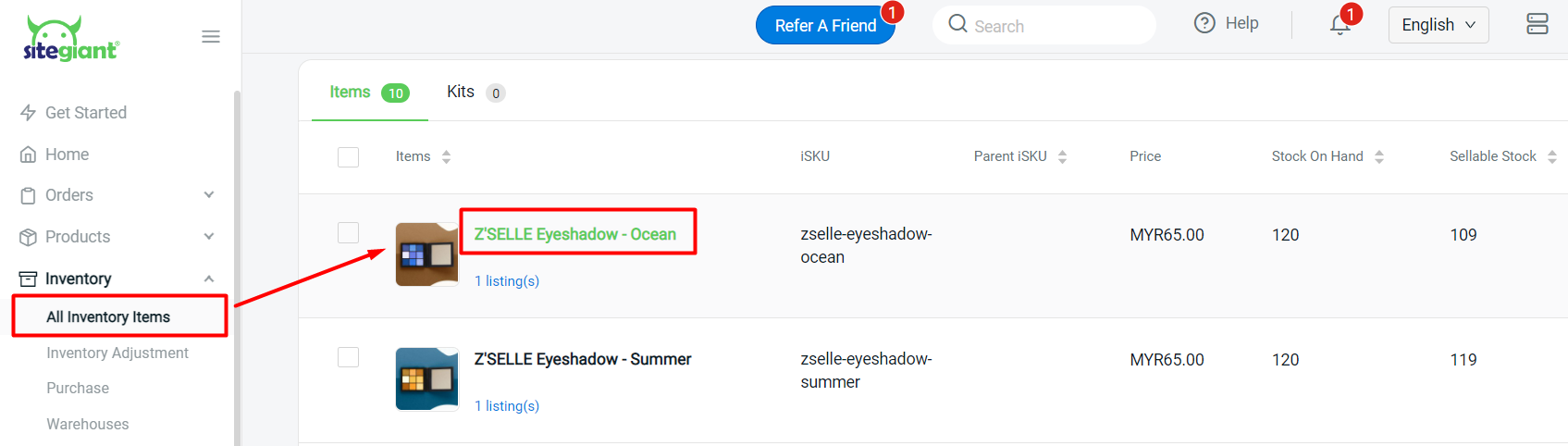This image showcases a screenshot from the 'Sight Giant' inventory management system. In the upper left, the logo displays 'Sight' in black and 'Giant' in green, featuring all lowercase, bold letters. Beside the text, there's a stylized demon head—a circular shape with two dots for eyes and two horns protruding from each side.

Under the logo, a navigation menu includes options such as 'Get Started,' 'Home,' 'Orders,' 'Products,' 'Inventory,' and 'All Inventory Items.' 'Inventory' is currently selected, displayed in bold text. Within the inventory menu, options like 'All Inventory Items,' 'Inventory Adjustment,' 'Purchase,' and 'Warehouses' are available, each accompanied by small icons. 'All Inventory Items' is highlighted with a red square, and an arrow indicates the first item on the list: 'Z-Cell Eyeshadow Ocean.'

A grid layout presents various makeup items, first showing 'Z-Cell Eyeshadow Ocean,' followed by 'Z-Cell Eyeshadow Summer.' Each product detail includes the SKU ('ISKU'), parent SKU, price (both listed as MYR 65), stock on hand (120 units for both), and sellable stock (109 for 'Ocean' and 119 for 'Summer').

Above the item list, additional interface elements include tabs for 'Items,' 'Kits,' and 'Refer a Friend,' along with a search bar, a help icon, an alert icon with a red number 1, and a question mark button.